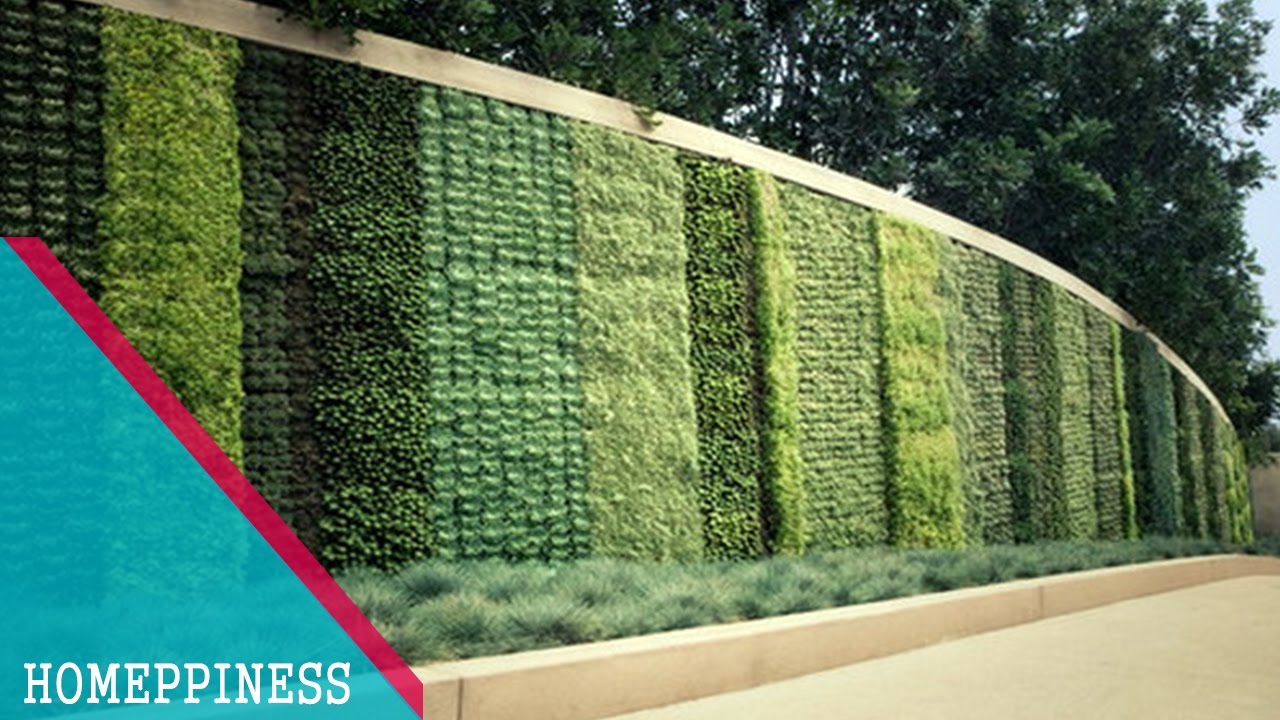In the image, we see a wall alongside a street, adorned with neatly groomed vertical patterns made of various green plants. These patterns range from light to dark green and are arranged in long, narrow columns that stretch across the entire wall. Some of the patterns are simple squares, while others take the shape of small dog-like figures. In front of the wall, there are short green bushes lining the curb, leading our eyes towards a rich background filled with dark green trees that obscure most of the sky. Notably, in the bottom left corner of the image, there's a blue triangle with a red diagonal stripe across it, containing the curious text "HOMEPPINES," a playful take on the word "happiness."